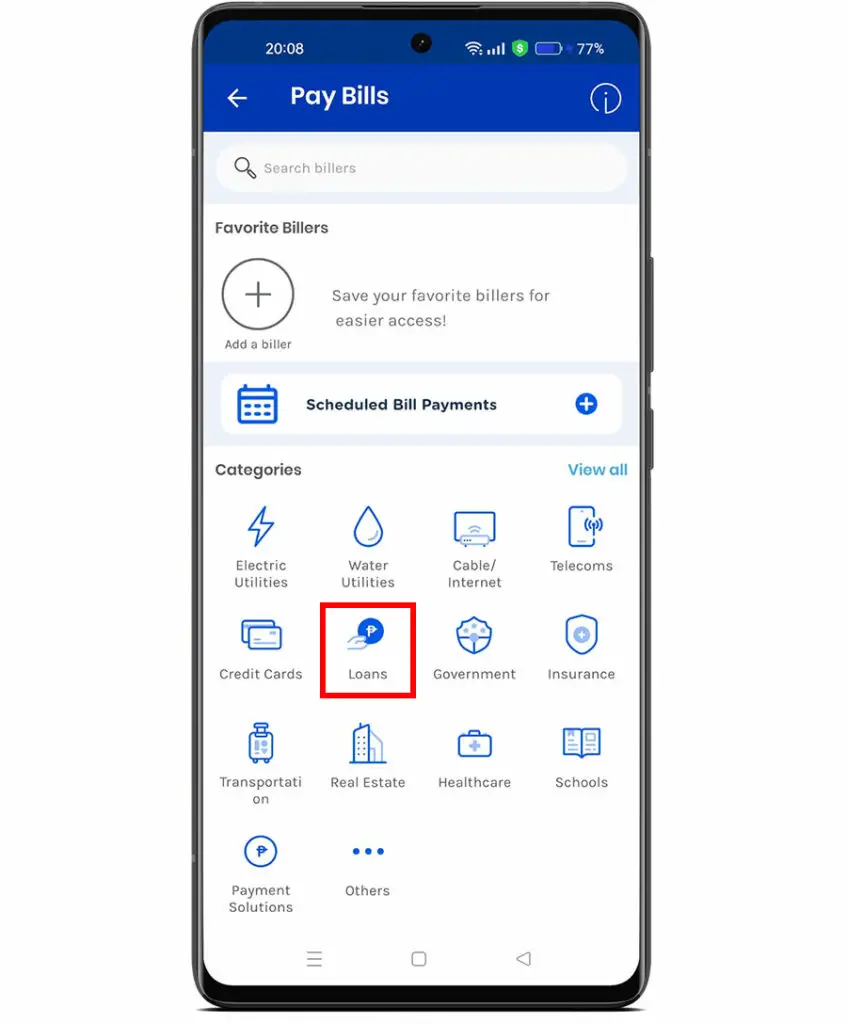This image captures the entirety of a black smartphone, showcased in an upright position. The edges of the phone are clearly visible, illustrating the physical design of the device. On the right side of the phone, the volume buttons are distinctly noticeable. The top left corner of the phone screen displays the time as "20:08." On the right side of the screen's topmost section, the Wi-Fi signal icon and the battery indicator are shown, with the battery at 77% charged.

A prominent blue banner sits at the top of the screen, emblazoned with the white text "Pay Bills" and a left-facing arrow. Directly below this banner is a search box containing a magnifying glass icon, designated for users to "Search Billers." As you scroll down, the section labeled "Favorite Billers" appears, offering an option to add favorite billers for quicker access.

Further down, a small calendar icon signifies the scheduled bill pay section, accompanied by a blue plus symbol for adding new scheduled payments. Following this section is a heading labeled "Categories" in black text. Below this are various categories, each paired with an icon. The category text is a grayish color, while the icons feature a blue hue. The listed categories include:

- Electric Utilities
- Water Utilities
- Cable Internet
- Telecoms

Following are categories for:

- Credit Cards
- Loans (highlighted with a red box to indicate selection)
- Government
- Insurance

The subsequent categories are:

- Transportation
- Real Estate
- Health Care
- Schools

The final line of categories includes "Payment Solutions" and "Others."

At the very bottom of the screen, navigation icons are displayed: three horizontal lines representing a menu, a square icon, and a play button icon.